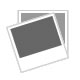The image depicts a small plush toy called Matokai, created by TS-PROS, Inc., encased in a clear, white mesh-like bag situated on a wooden surface with a light yellow background. The toy, resembling a quirky, black, rabbit-like creature, features a round head with long ears standing upright, each adorned with subtle gray markings. The plush has large white oval eyes, with one eye partially obscured as the head is slightly turned to the right. Covering its mouth is a red mask that extends under its jaw up to the nose area. The toy is dressed in a white t-shirt emblazoned with a red grenade emblem and complemented by red sleeves. Its hands and legs are also black. The packaging has a black rectangular label at the top, which reads "Matokai" in white lettering, with additional, unclear white writing beneath it.